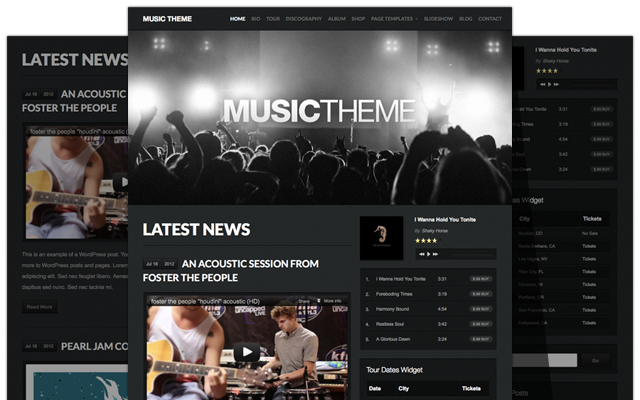The image showcases a digital layout of a rock music-themed website with a predominantly black and dark gray color scheme. The topmost section prominently features a page titled "Music Theme", which is dominated by a striking black-and-white photograph of a lively crowd at a concert, with stage lights illuminating the scene from a distance. Below this main section is a segment labeled "Latest News", followed by another section dedicated to an acoustic session by the band Foster the People. Here, a vibrant, color image of a few musicians performing is displayed, which is actually a clickable video link leading to further content. Adjacent to this video link is a section providing tour date information for Foster the People. The larger, underlying window beneath this top layer features an extended content page that offers more detailed information, including a mention of Pearl Jam and what appears to be concert dates and locations, possibly indicated by the abbreviation "CO".